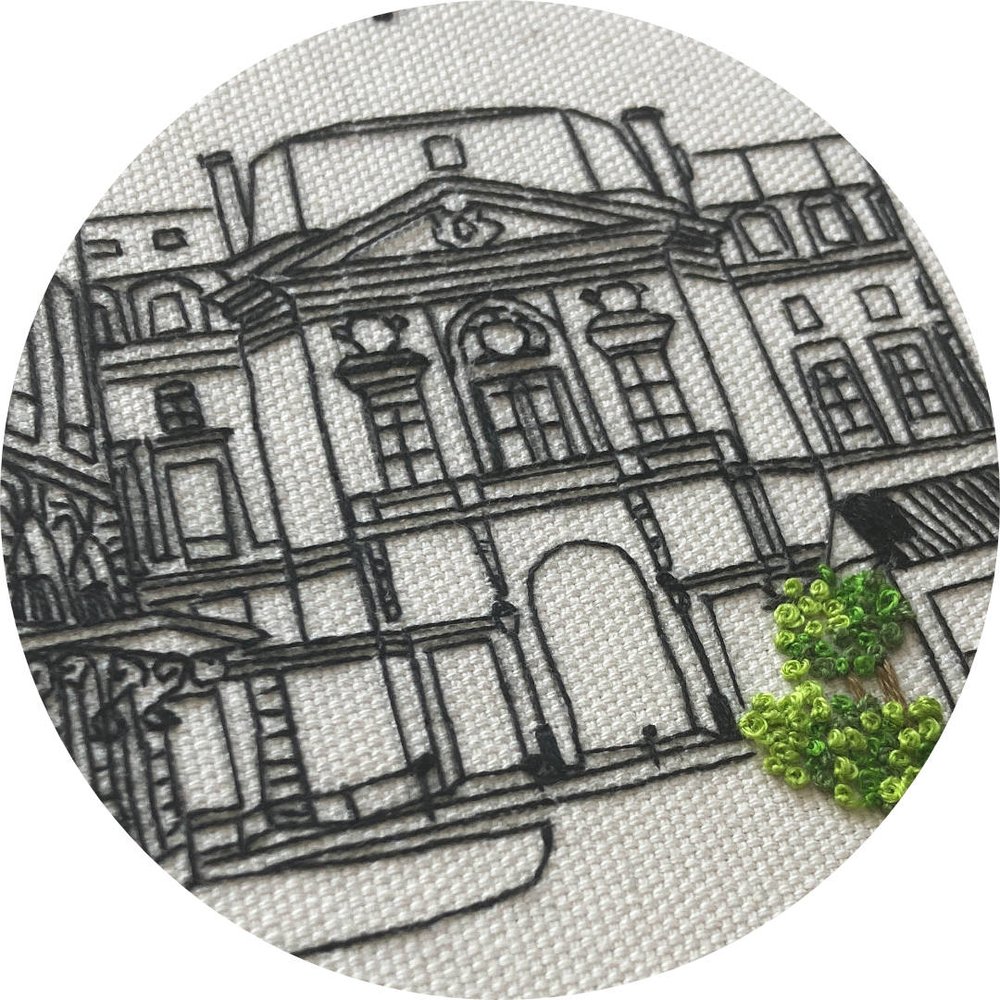The image captures a detailed needlework or embroidery on a white, tightly woven fabric sheet, viewed from an overhead angle. The artwork itself is circular and features the outline of an old, multi-story house made with fine needle line work on black fabric. The house, which has an arched doorway and numerous windows, exhibits a historical aesthetic. In the lower right corner, there is a small shed accompanied by a three-dimensional green tree. The tree is intricately crafted with thin brown trunks and circular leaves, creating a realistic effect.